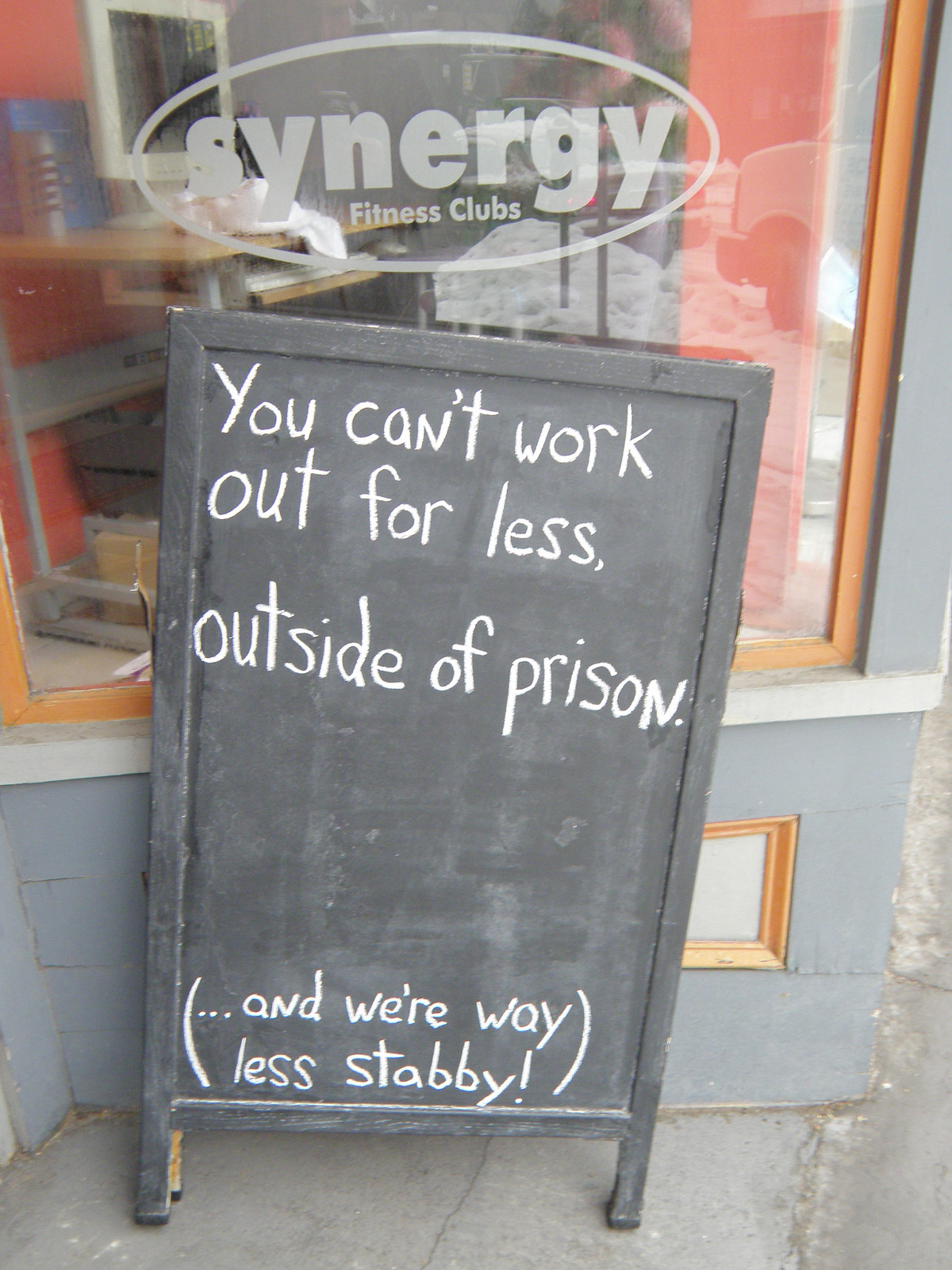The photograph captures the exterior of Synergy Fitness Clubs, prominently featuring their logo in the glass window. In front of the building, which is painted light blue with gold and white trim, rests a blackboard sign placed on the sidewalk. The sign, written in white chalk, humorously states, “You can’t work out for less outside of prison,” and adds in parentheses at the bottom, “and we’re way less stabby!” This chalkboard advertisement, advocating the fitness club's low prices with a playful prison reference, stands just below the club's logo in the window. The interior of the fitness club is somewhat obscured, but a glimpse of a table set with a white computer monitor and keyboard is visible through the glass.